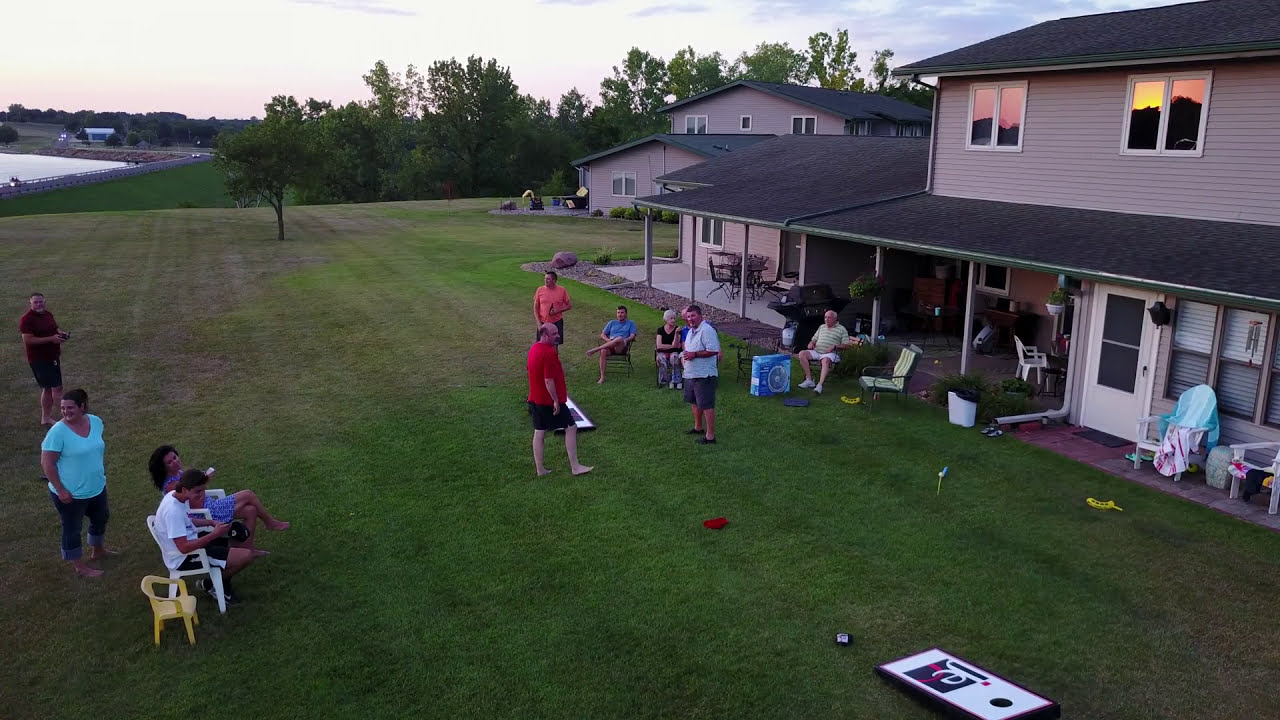In this photograph, a backyard get-together unfolds in a spacious, unfenced grassy area flanked by connected residential homes. The central focus is a tan, two-story house with two sets of second-story windows reflecting a stunning sunset of red, orange, and yellow hues, creating an illusion of a mountainside. The house features a white back door near which a chair draped with towels sits. Scattered across the lush green lawn, clusters of people engage in socializing and activities. 

Three men stand in the middle of the yard participating in a cornhole game, their beanbags strewn on the grass. One man, in a white shirt and dark shorts, interacts with another man wearing a red t-shirt and black shorts, who is barefoot. Nearby, several women lounge in white plastic lawn chairs, observing the game and chatting. Among them, a woman in a blue dress with dark hair smiles at a younger man in a white t-shirt and shorts seated next to her.

To the left, a woman with brown hair in a ponytail, clad in a blue t-shirt and blue jean capris, smiles while looking off-camera. Standing behind her, an older man with a red t-shirt, shorts, a beard, and very short hair also watches the scene, barefoot like the others. Through the background trees, hints of a lake or pond glisten. Another two-story tan house peeks from behind the main house on the right, completing the serene and communal atmosphere of this sunset-lit gathering.